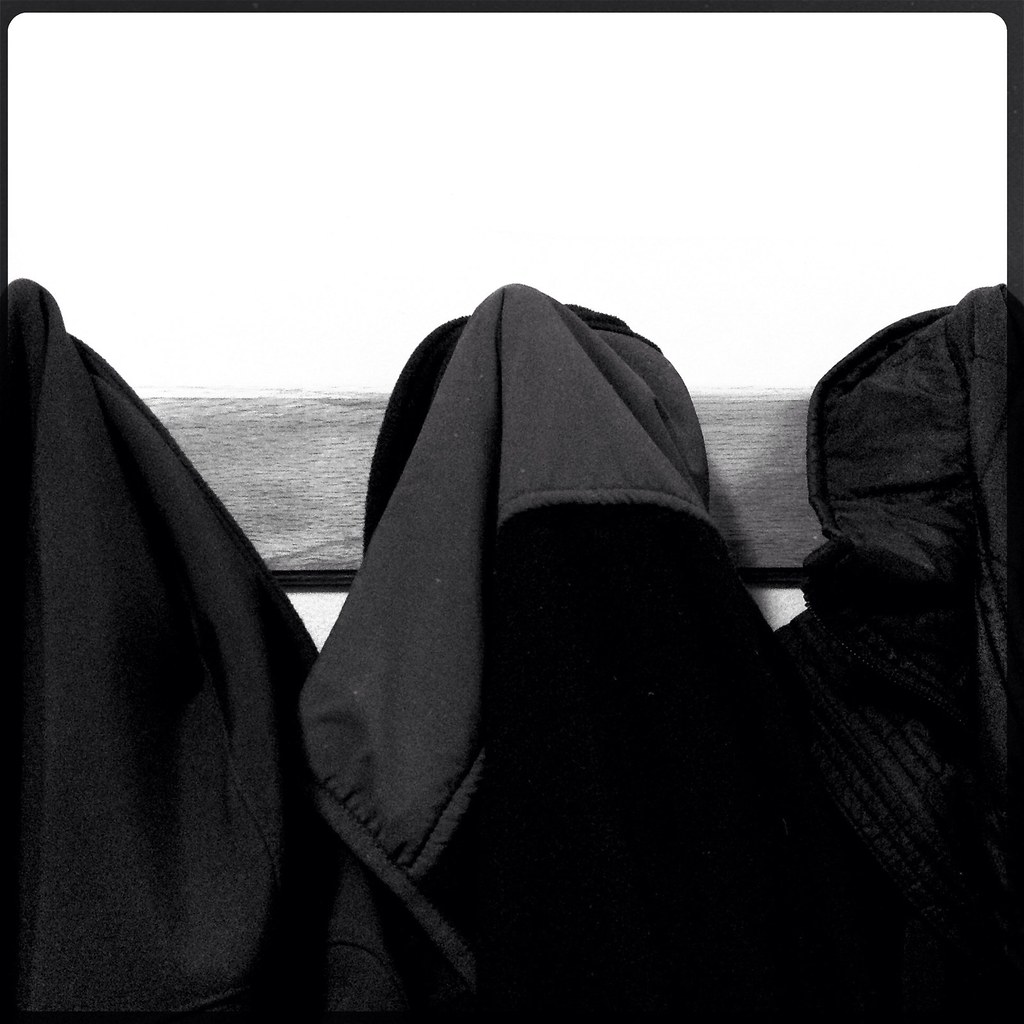The image depicts a high-saturation, black-and-white photograph featuring three black coats hanging on large hooks attached to a horizontal wooden plank, likely a 2x4. These coats are aligned against a stark white wall. The edges of the photograph are marked by a slight black outline. Each coat showcases different textures: the leftmost coat has a sleek, cloak-like appearance, the one in the middle appears to have a lighter black section and a hood folded over a hook, while the coat on the right has its fabric wrapped in a turban-like shape. The wooden plank contrasts with the wall, creating a clear separation, and the bottom of the image appears predominantly black, enhancing the coats' visibility.